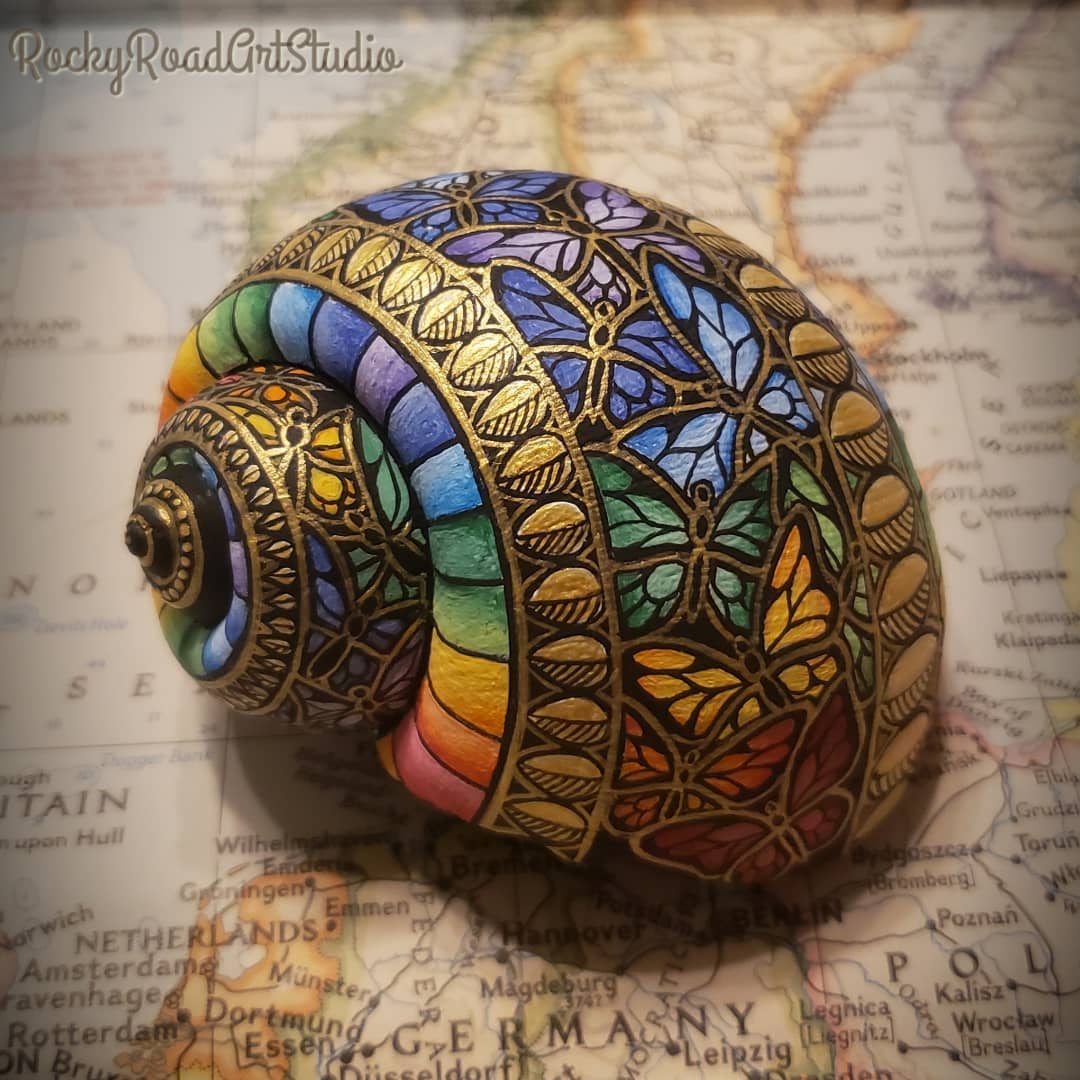This image features a vividly decorated snail shell set against a map of Europe. The map, rendered in muted tones of orange, green, tan, and red, clearly shows regions like Germany and Poland, though they fade into the background, directing focus to the art piece. The upper right-hand corner of the image bears a cursive watermark that reads "Rocky Road GRT Studio."

At the center of the image, the snail shell itself captures attention with its intricate design, resembling stained glass. The shell's structure follows a traditional coiled pattern, reminiscent of a cinnamon roll, spiraling inward. The outer edges boast a rainbow spectrum, with bold black lines marking transitions between colors. Strips of black background adorned with gold leaf motifs encircle the shell, adding to its ornate appeal.

In the core of the shell, gold-outlined butterflies in rainbow hues draw the eye. Alongside these butterflies, the shell's design also includes elements reminiscent of seeds or cowrie shells, surrounded by detailed borders, swirling circles, and decorative filigrees and dots, all contributing to its elaborate and striking appearance.